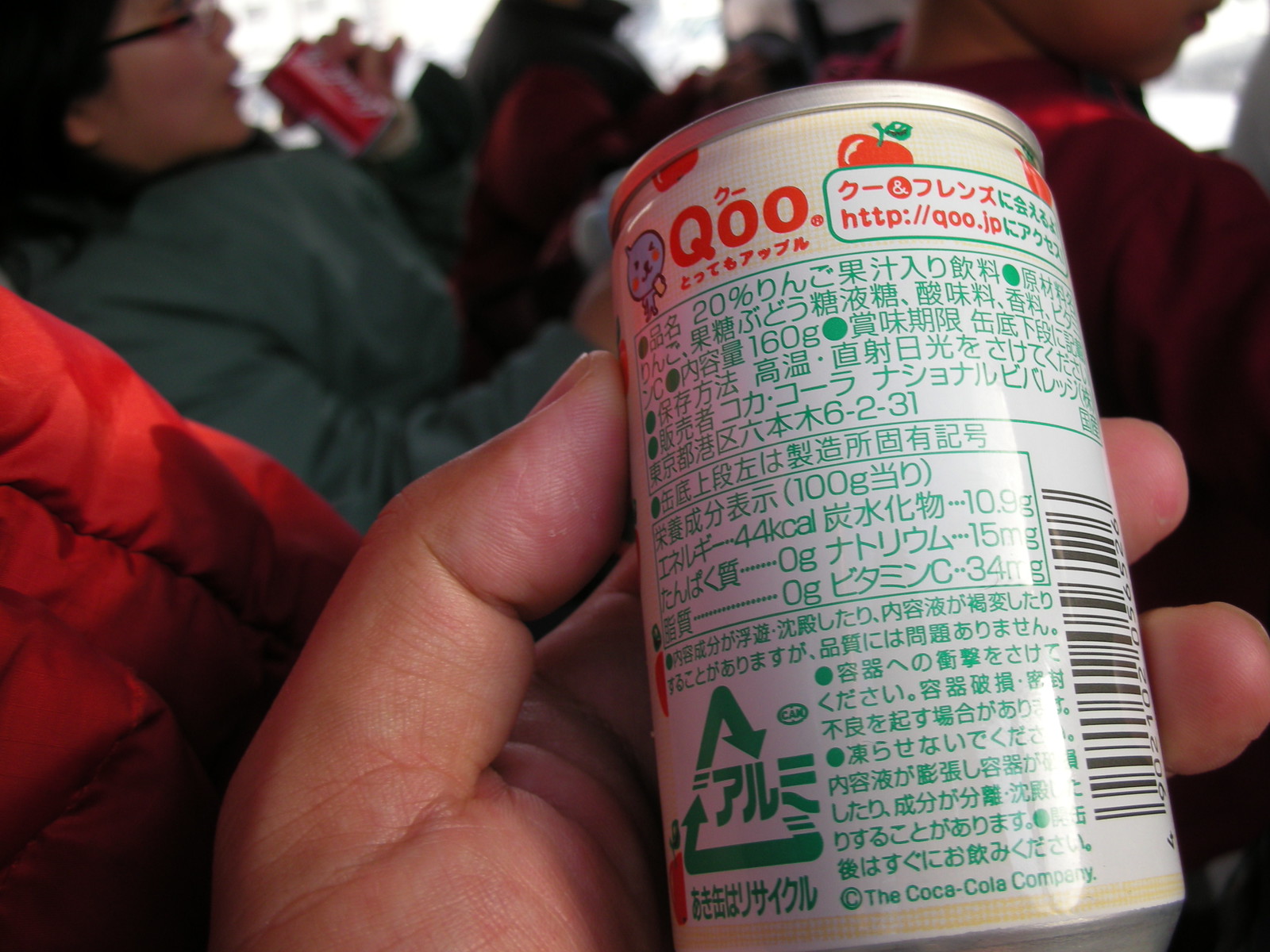The image captures a close-up of a small, cream-colored aluminum can, resembling a mini version of a regular Coke can, held in someone’s left hand. The person's thumb and two fingertips securely grip the can, which features a silver top and various intricate graphics. Prominent on the can is a blue circle with a cartoon face – two black eyes, a black nose, and a smiling mouth with red cheeks. Surrounding it are graphics of apples, complete with stems and green leaves, and Chinese writing, hinting at its Asian origin. Notably, the can bears the text "QOO" as a registered trademark, and at the bottom, it reads "The Coca-Cola Company" with a small box displaying the URL "HTTP://QOO.JP." There's a visible barcode on the back. In the background, partially cropped out, is an Asian woman with dark hair, glasses, and a green long-sleeved sweater. To the left of the hand, another person in an orange jacket is faintly visible. This detailed scene is set among a group of people, emphasizing the can’s unique design and cultural elements.